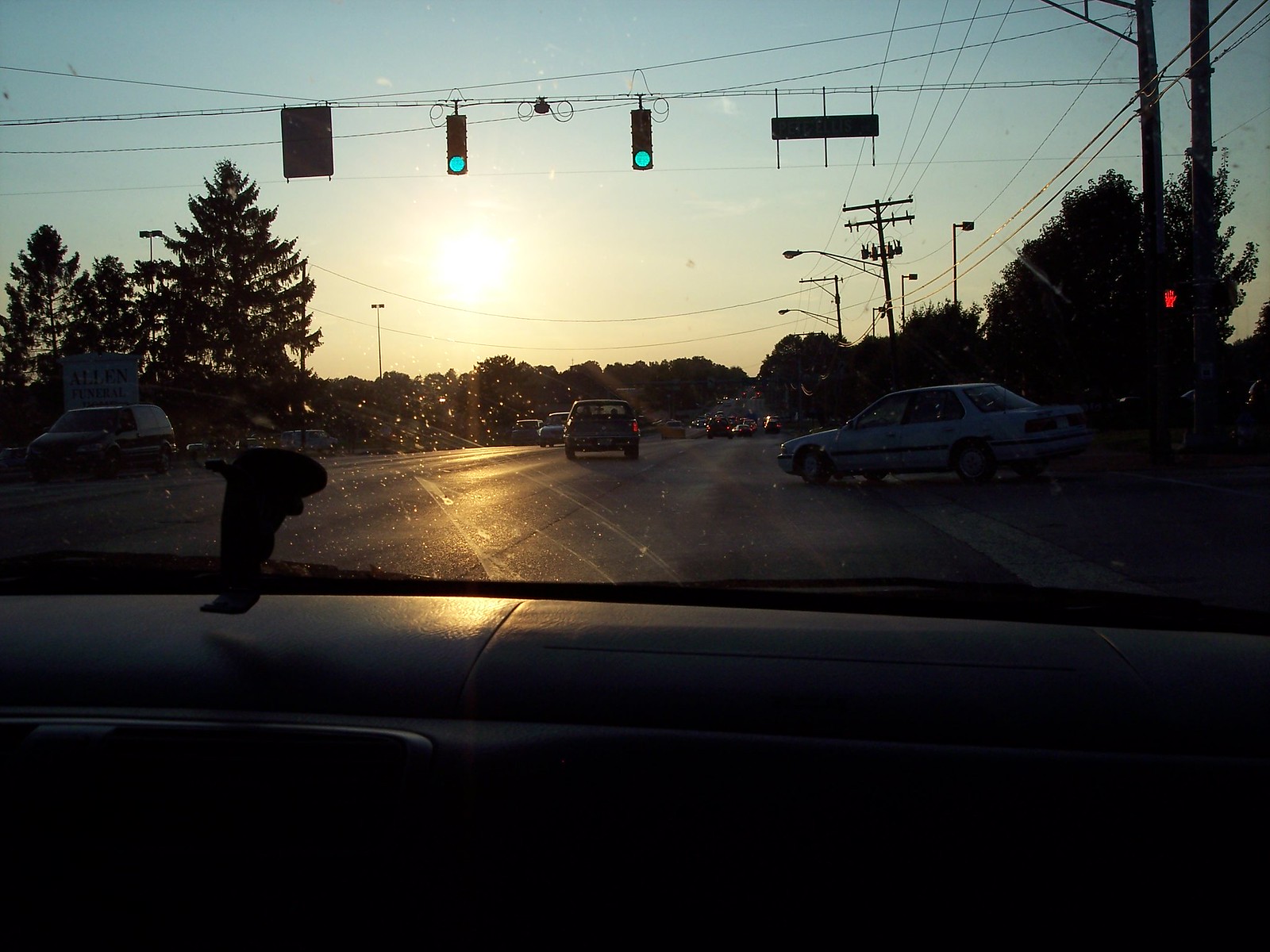The photograph, taken from the passenger seat of a car, captures a vivid scene at an intersection. The image, though primarily in color, shows distinct aesthetic details with a mix of light and shadow. There's a low, bright yellow sun near the horizon that lights up a blue sky partially covered with clouds, casting a beautiful streak of sunlight on the asphalt road while the rest remains dimly lit. Power lines and light poles stand along the street, with two green traffic lights hanging above. From the dashboard with black leather, sunlight reflects faintly, also revealing a dashcam. The scene is bustling with vehicles – some waiting at the intersection, others including a white sedan making a right turn, and cars with taillights on moving in both directions. The adjacent crosswalk displays a red hand for stop. Farther in the background, you can see trees lining the streets but obscuring any buildings, adding to the overall serene yet lively atmosphere.